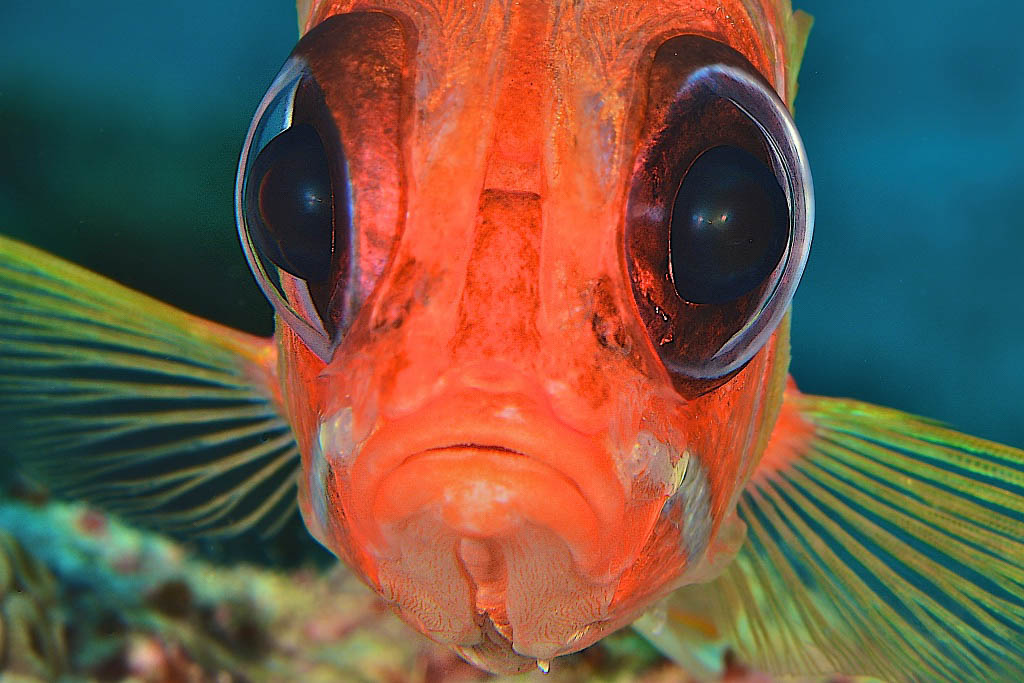This image is a close-up of an orange fish, likely a goldfish or some variety of carp, prominently filling the frame of a wide vertical rectangular image. The fish's large, bulging black eyes, covered with clear lenses, are staring straight at the viewer, giving it a very direct, almost comical appearance. The background is somewhat blurred but shows medium to dark blue water, suggesting the fish is in an aquarium setting. Below the fish, there are indistinct colors and shapes, potentially gravel or rocks in brown and red hues.

The fish's primary color is a vivid orange, with touches of white just above the lips on either side of its slightly frowning mouth, which appears almost cleft along its chin. The fins on either side of its face start as a pale yellow at the base and transition to a deeper orange. There is also a yellowish color noticeable behind its bulging eyes. This yellow coloring might also be present along the fish's side, although it is not distinctly clear due to the blur. Overall, the detailed focus on the fish's face and features creates an engaging and vibrant portrait of this aquatic creature.